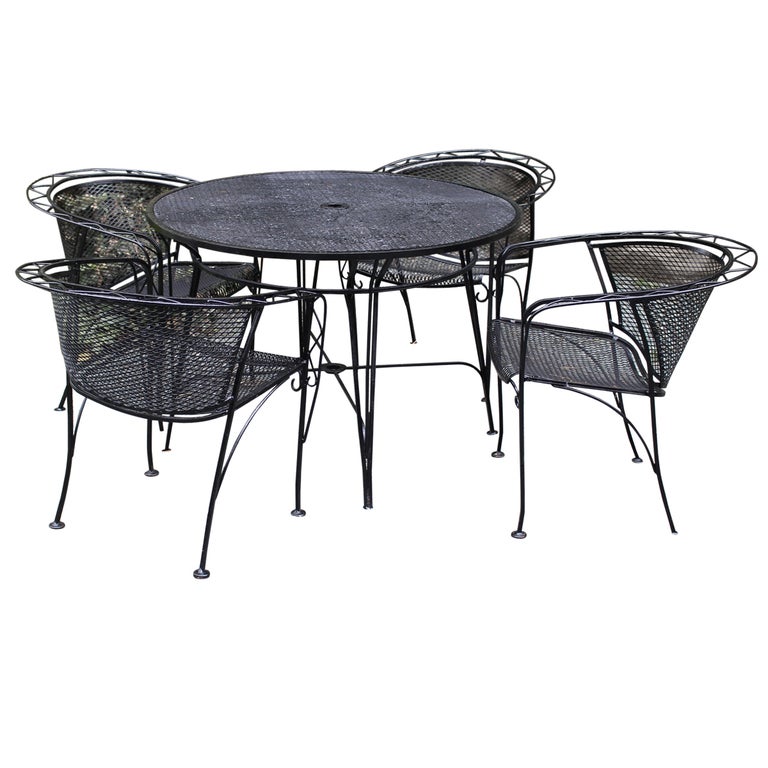This photograph showcases a black iron outdoor patio set against a clean white background, possibly for an online product advertisement. Central to the image is a circular table with a small hole in the middle designed for a parasol umbrella. The table stands on four thin, wiry legs with connecting supports near the base. Surrounding the table are four identical chairs fashioned from the same black metal material. Each chair features a mesh-patterned backrest and seat, and they are characterized by their slender legs that converge into circular bases. The backs of the chairs have a singular wire line pattern at the top, and they possess a subtly curved line that extends from the arms around the back to the front. Despite the otherwise transparent background, there is a minor flaw where the image wasn’t fully photoshopped out correctly, adding to the realistic depiction of the furniture set.